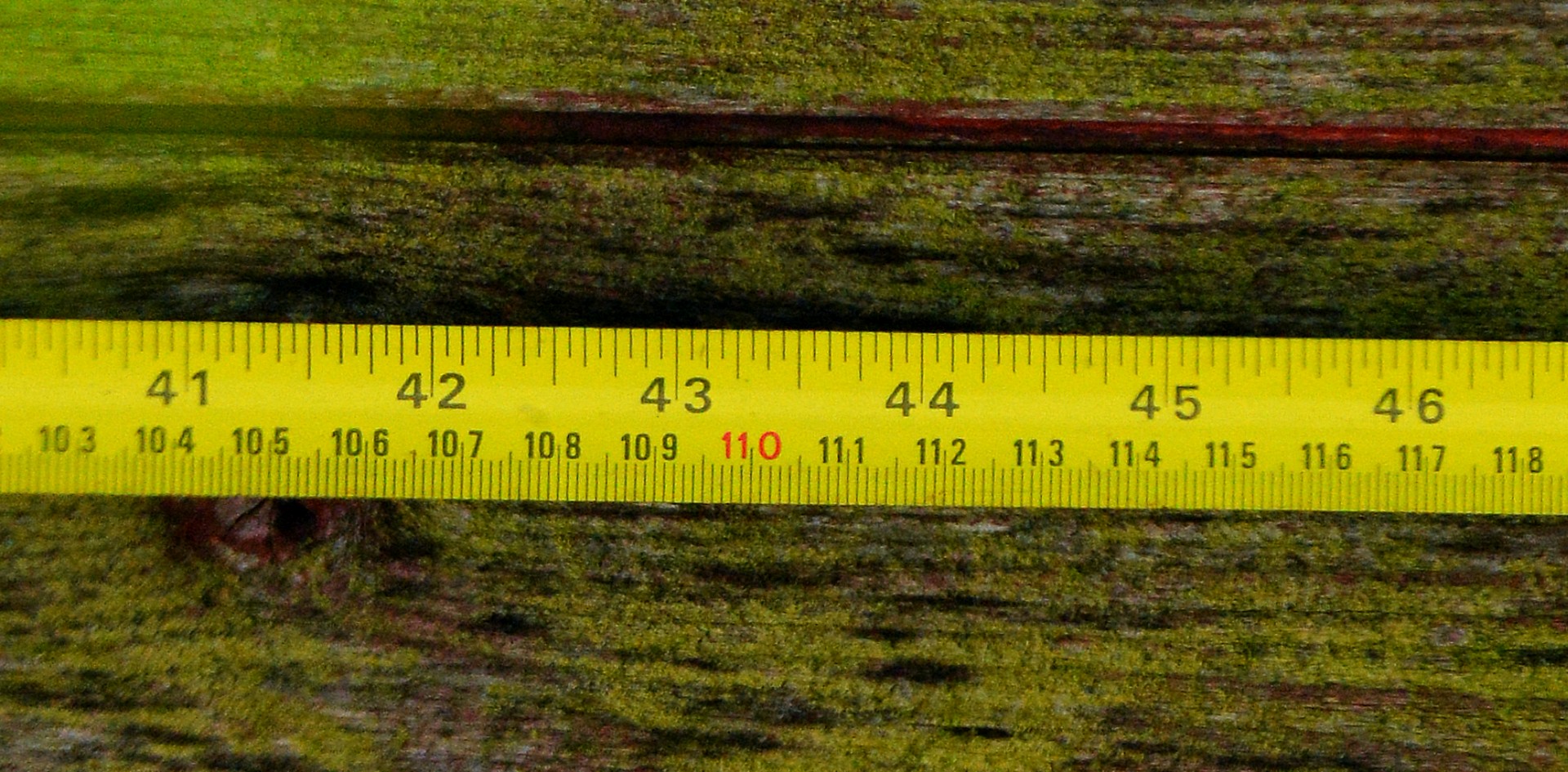This color photograph captures a close-up view of a yellow retractable tape measure laid horizontally across an old, dark wooden table. The visible portion of the tape measure spans from the 41-inch mark to the 46-inch mark, with corresponding metric measurements from 103 centimeters to 118 centimeters. The frame of the photograph is approximately seven inches wide, tightly cropping the scene to focus solely on the tape measure and the textured wood grain beneath it. The image is presented in landscape aspect ratio, making it wider than it is tall, with no people, animals, plants, buildings, or mechanical objects present.